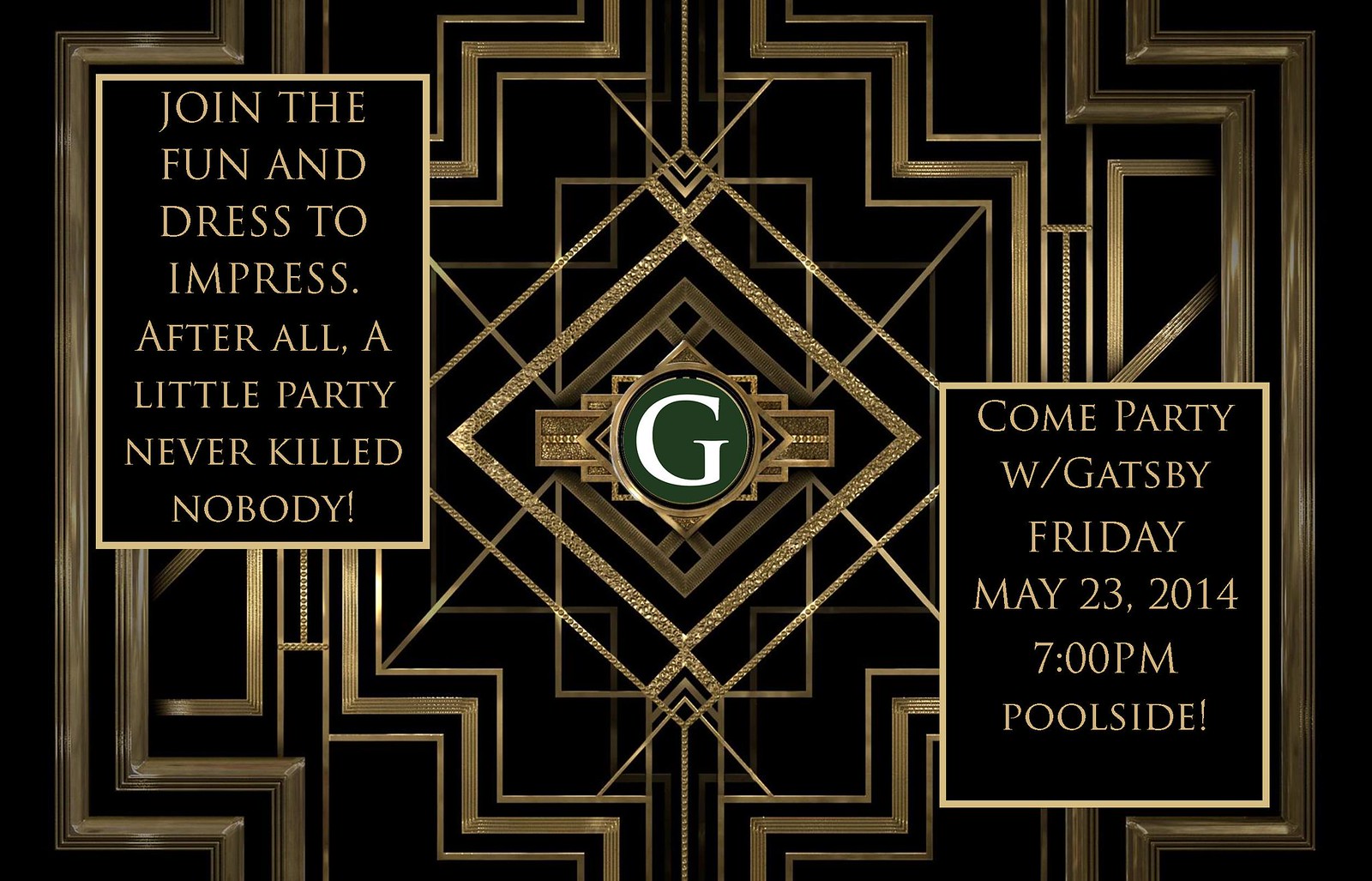The image features an elegant black and gold sign with a distinctive emblem at its center. The emblem consists of a capital letter "G" encircled by a green circle, overlaid with white text. The sign's main body bears the inviting message: "Join the fun and dress to impress. After all, a little party never killed nobody." Below this, in the bottom right corner, a smaller gold-bordered box contains additional event details: "Come party with Gatsby, Friday, May 23rd, 2014, 7 p.m., poolside."

The design includes intricate detailing, highlighted by a sophisticated, royal gold and black logo featuring a central diamond shape, outlined by another diamond. This luxurious theme is further emphasized by fine gold lines that frame the entire image, adding a touch of grandeur and refinement.